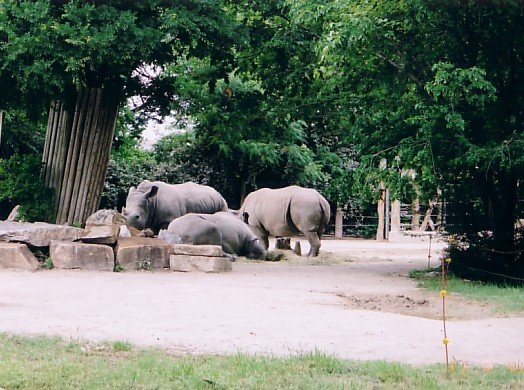In this detailed and somewhat aged photograph, likely taken with an older or disposable camera, we see three rhinoceroses in an outdoor habitat enclosure, possibly at a zoo or a reserve in Africa. This dirt and gravel clearing is framed by lush green foliage and tall trees, lending a sense of wild natural beauty. Among the noticeable features is a wire fence in the background, with portions visible on the right side, and a sturdy pillar adorned with smaller branches. The immediate environment of the rhinos includes scattered rocks and mounds of dirt. The rhinos themselves are positioned distinctly: one lays down resting, another stands behind facing to the left, and the third stands slightly behind and to the right, facing away. Despite looking like they're just relaxing, these majestic creatures remain the focal point of the image, juxtaposed against the vibrant greenery and modest surroundings of their enclosure.